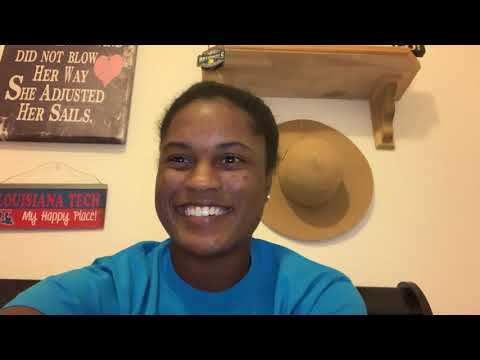In the center of the image sits a young black woman with short black hair and a radiant smile, her top teeth visible. She is wearing a light blue t-shirt and appears to be indoors, possibly engaged in a live stream or video call, looking slightly off to the left of the camera. The background features various objects and decorations: to the top left, there are a couple of pictures and a small shelf with an unreadable hang sign. Further to the left, a tan hat hangs on the wall. Prominently displayed on the wall are two signs; the upper one, with white text on a black background, reads, "Did not blow her way. She adjusted her sails." Below it, a pink card accents the top right corner of a black placard that says "Louisiana Tech" with the subtitle "my happy place" and a small symbol to its left. The setting suggests it is midday, with the scene exuding a cozy and personal atmosphere. The image is vibrant with colors such as brown, white, pink, blue, red, light blue, tan, and black.